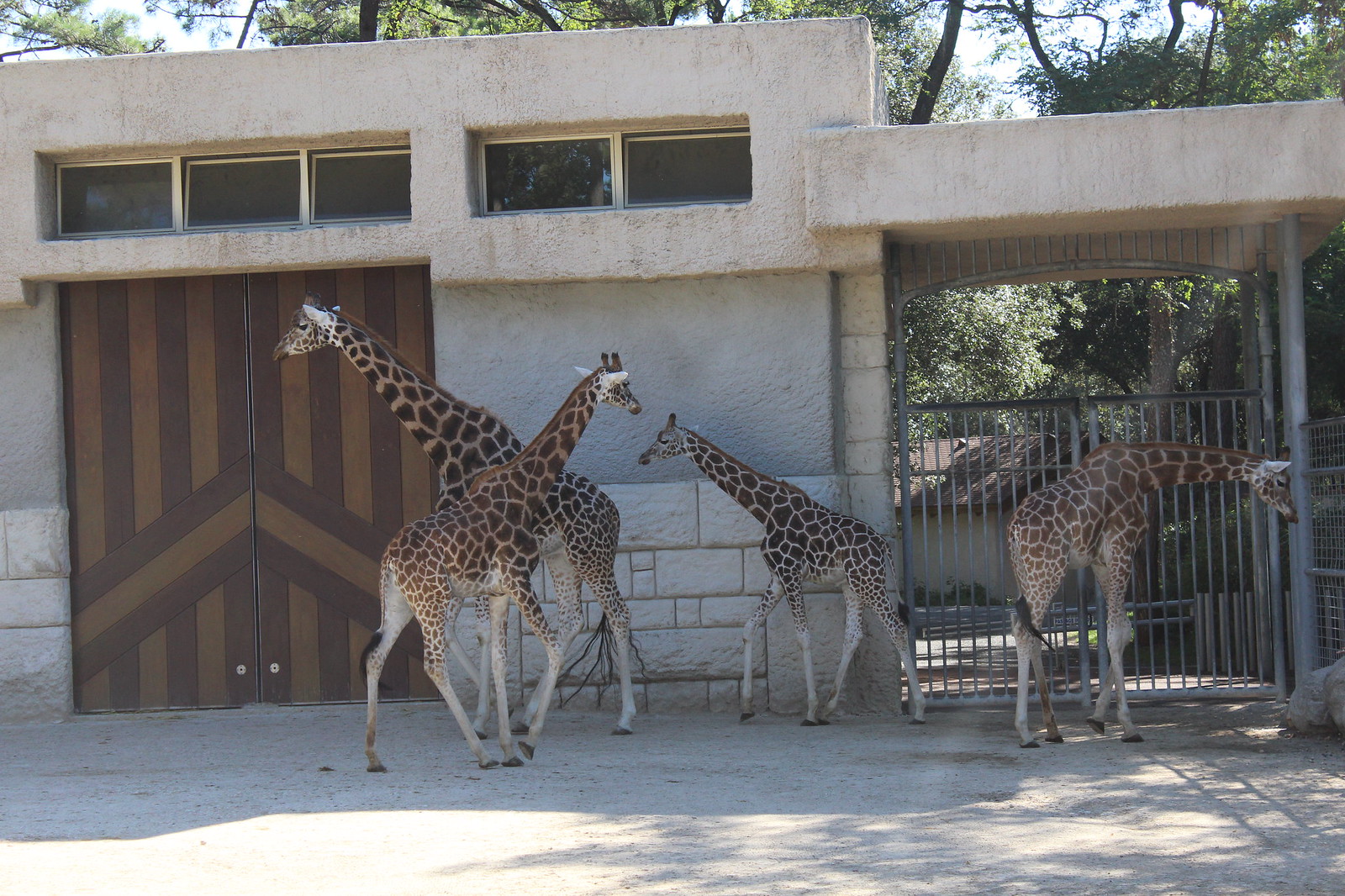This horizontal color photograph, taken outside on a bright sunny day, depicts a zoo enclosure bathed in pastel and red toned lighting. Central to the image is a stucco cement building adorned with five rectangular windows at the upper part and distinct brickwork at the lower portion. Dominating the structure is a tall, striped dark brown and light brown door, presumably used for the giraffes to move in and out.

In the forefront, four giraffes, likely of the reticulated variety, occupy the enclosure. The two adult giraffes stand to the left center, facing or angled sideways, while two juveniles stand to the right, each oriented in opposite directions. The tallest giraffe, positioned towards the back left, has a smaller one just behind it. In front of the tallest giraffe, another giraffe faces right, sharing the same head angle as those to its left. However, the fourth giraffe, situated on the far right, has its head positioned level with its back, appearing as if it is looking down.

The enclosure itself features a cement ground with dappled sunlight filtering through surrounding trees, creating spots of light and shadow. To the right, a metal gate or fence leads into a covered area attached to the building, completing the secure confines designed for the giraffes. The photograph captures a serene moment in the giraffe enclosure, with detailed attention to both the animals and their habitat.